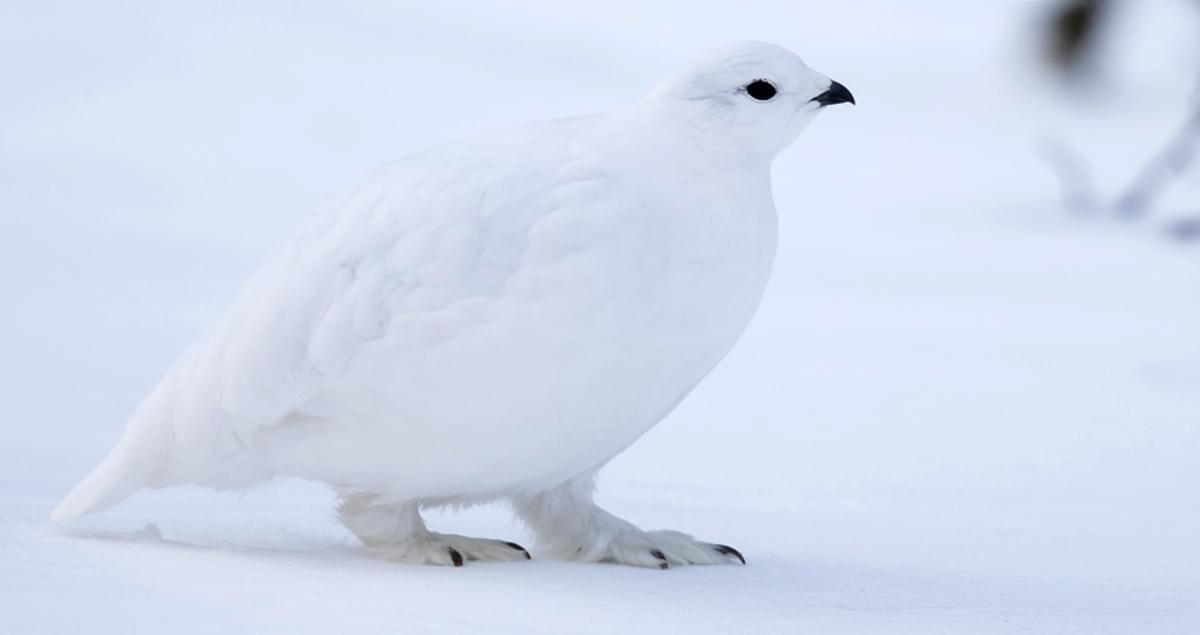This captivating photograph showcases a beautiful, pure white bird standing on a snow-covered ground, against a backdrop that's slightly blurred to a white hue, indicative of the cold, natural environment. The bird is depicted in a right profile with its small, beady, black eyes and a tiny, black beak. The entirety of its body is covered in densely packed, furry-like feathers that give it a very plush appearance. Its feet, just as furry as its body, have distinct black claws. The bird is somewhat plump with a substantial body and white tail feathers. There is a faint black element in the upper right corner of the image, but the scene is predominantly white, accentuating the bird's striking monochromatic plumage. The overall composition and serene ambiance resemble a high-quality photograph one might find in a nature magazine like National Geographic or an exquisite snapshot taken by a birdwatching enthusiast.